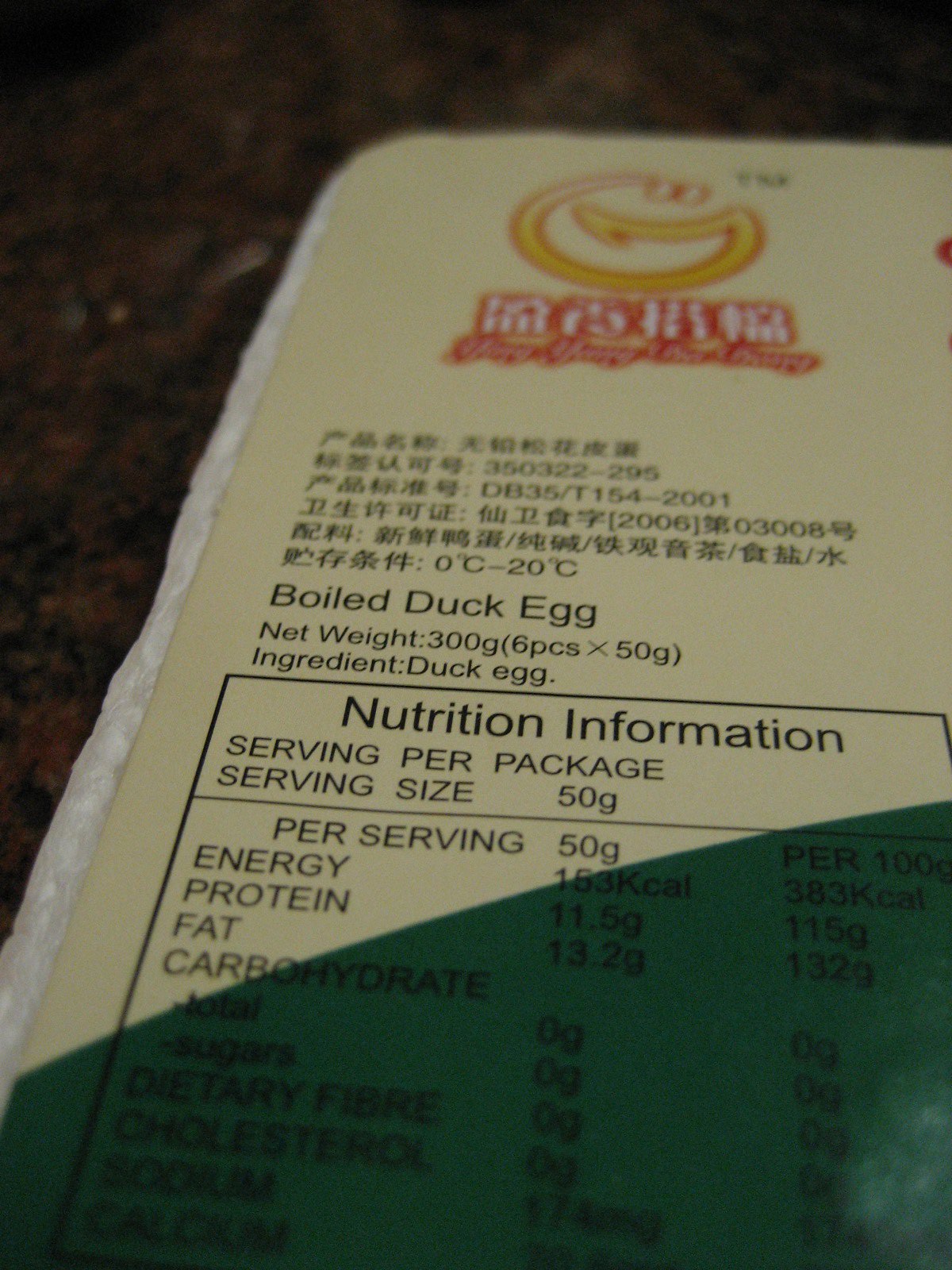This vertically oriented, blurry, low-quality color photograph captures the label of a boiled duck egg package, positioned upon a table. Dominating the top of the label is a partially visible logo, embellished in red and yellow, although the details are indistinguishable. Beneath this logo, an array of Asian language characters spell out "boiled duck egg." Further down, the label features a nutrition information section, outlined in black, and filled with text detailing serving size, energy, protein, and fat content. A prominent dark spot or shadow with a greenish hue diagonally intrudes upon the bottom portion of the image. The photograph appears to have been taken under artificial lighting, with the package resting on a table, while the background reveals a reddish-brown carpet in the distance. The label overall is imbued with a greenish-yellow tint.